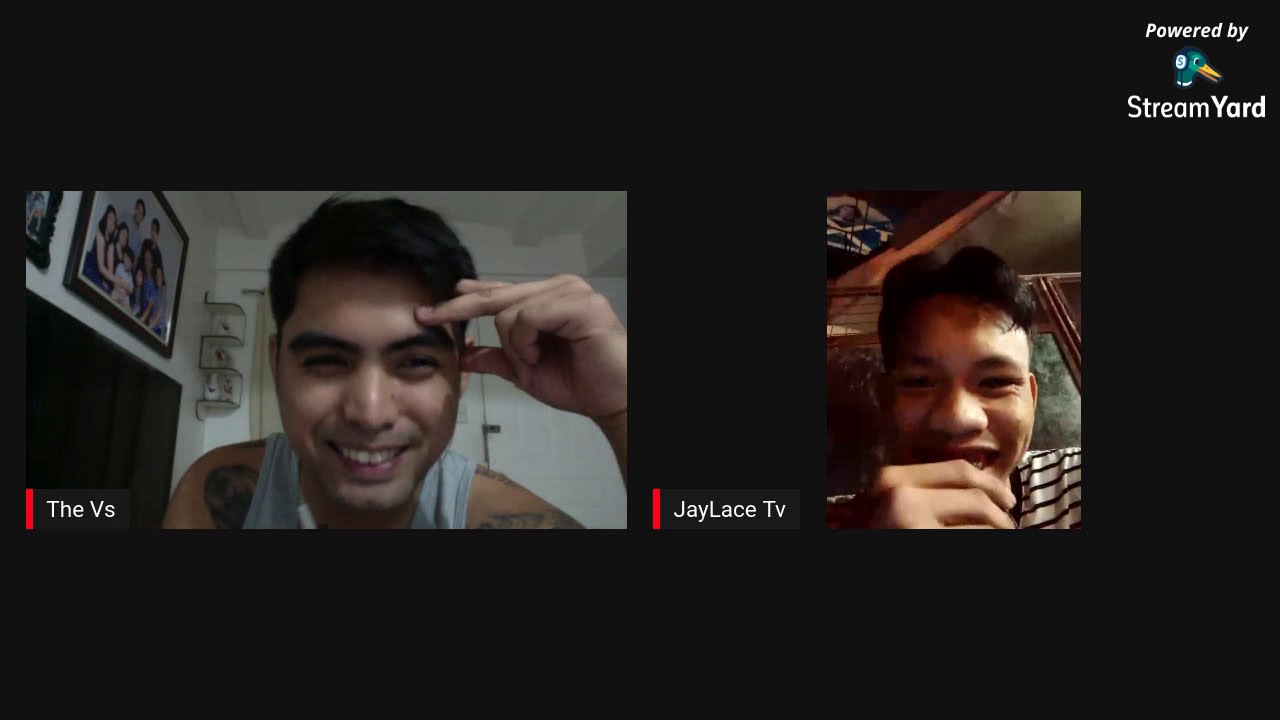The image presents a dual-stream setup with two young men, appearing as if on a Zoom call, set against a completely black background. In the top right corner, there's white text reading "Powered by StreamYard," accompanied by an image of a mallard duck with a green head and yellow bill, wearing headphones. 

On the left, a young man, likely in his late teens or early 20s, is shown in a larger rectangle. He has dark hair, bushy eyebrows, and is smiling broadly, revealing his upper teeth. He wears a white sleeveless t-shirt that showcases tattoos on his shoulders. His left hand is poised at his forehead with his thumb, index, and middle fingers touching his brow. In the background, family portraits are visible on the wall, suggesting he is at home. Text at the bottom left of his screen reads "The Vs."

On the right, a younger teenage boy appears in a smaller square. His face is partly obscured by his hands, with his fingers resting near his lips, and he is also smiling. He wears a white shirt with thin horizontal black stripes. Next to him, the text "J Lace TV" is displayed. The background is entirely black, contrasting with the setup on the left side.